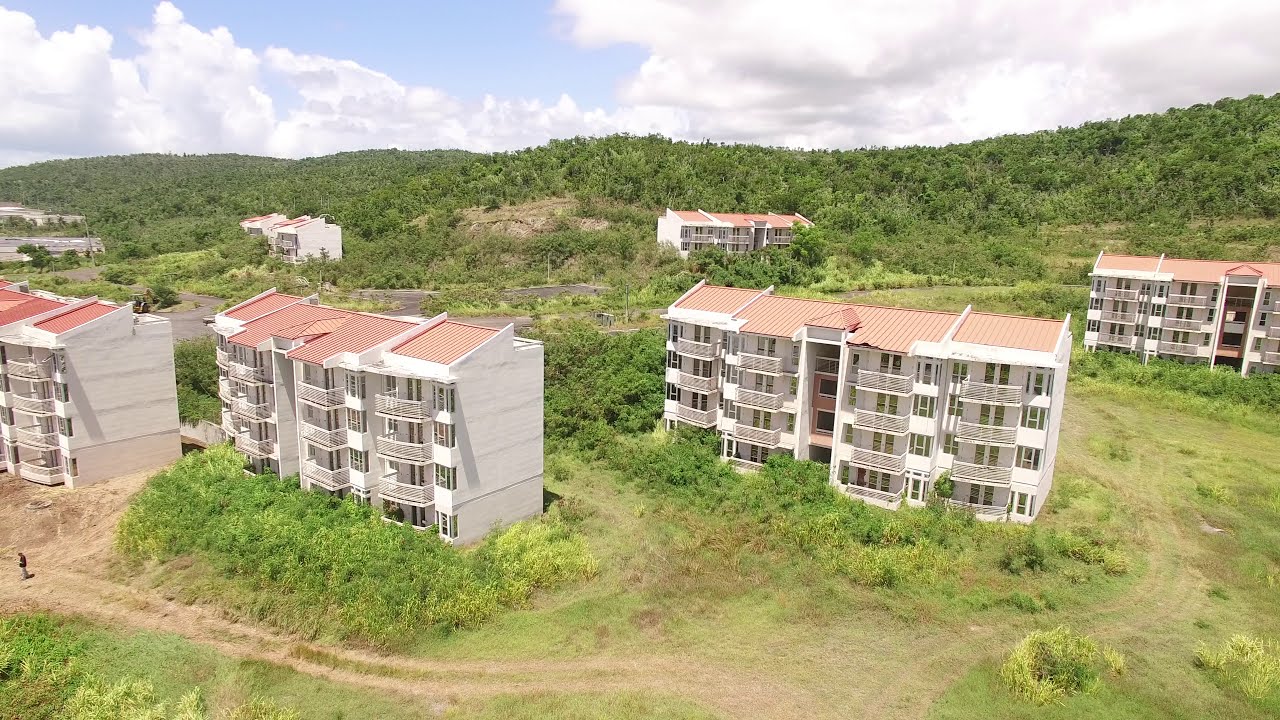The image is an aerial shot taken a few hundred feet above a remote area on a sunny day. In the upper quarter of the picture, the bright blue sky is dotted with thick white clouds to the left and right. Below the sky, a hillside covered with lush green shrubbery can be seen. In the foreground, there are six large buildings, each four stories high with reddish-orange, slightly sloped roofs that display subtle variations in pattern and color. Each building is divided into units, featuring balconies on each floor - four balconies across and four high. Dirt paths and overgrown greenery separate these buildings, adding to the scene's rustic charm. Despite their somewhat worn-out and poorly constructed appearance, there is an absence of scattered trash, lending an odd sense of tidiness to the otherwise impoverished structures. The background transitions into a wild hilly area, encapsulating the secluded nature of this setting.